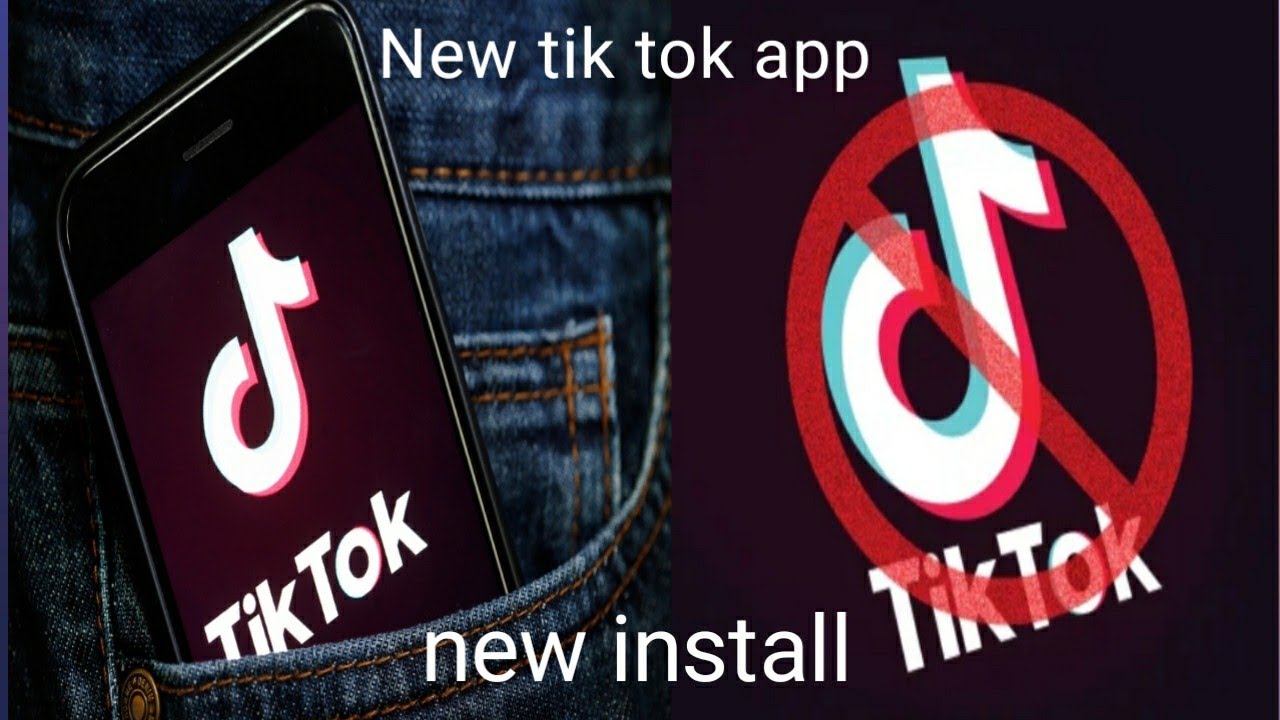This digital image prominently features a promotional banner for a new TikTok app. At the top of the image, the words "New TikTok App" are displayed in a sleek white font. The centerpiece of the image is a close-up view of someone wearing blue denim jeans, capturing only the lower back portion and the front pocket of the jeans. The gender of the individual is not discernible from the image.

The denim jeans are adorned with distinctive gold stitching around the front pocket. Nestled inside this pocket is a smartphone, with its screen clearly visible. The screen displays a TikTok logo accompanied by the word "TikTok" in white font. Positioned to the right of this logo is another TikTok icon, this time encircled in red with a diagonal line striking through it, indicating some form of prohibition or restriction. At the bottom of the image, the phrase "New Install" is written, suggesting a call to action for viewers to download or update the TikTok app.